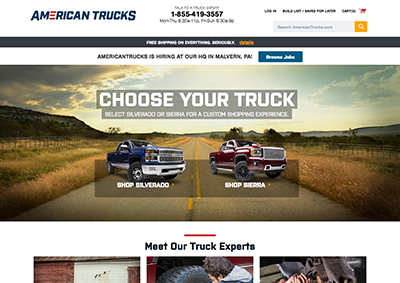The image showcases a screenshot from the American Trucks website. At the top, a prominently displayed phone number invites visitors to call for more information. The main banner features two trucks on a road with the headline "American Trucks is hiring at our HQ" located in Malvern, PA. Below this notice, detailed text highlights job opportunities and encourages users to choose their truck for a custom shopping experience.

On the left side of the page, a vibrant blue truck is featured alongside the caption "Shop Silverado." On the right side, a striking red truck is emphasized with the caption "Shop Sierra." Additionally, just beneath these sections, there's a call-to-action titled "Meet Our Truck Experts," accompanied by three photos of team members.

At the very top of the page, there's a search bar featuring a white magnifying glass icon within a distinctive yellowish-orange square, enabling users to quickly find products or information. This comprehensive layout aims to deliver a user-friendly and visually appealing shopping experience for truck enthusiasts.